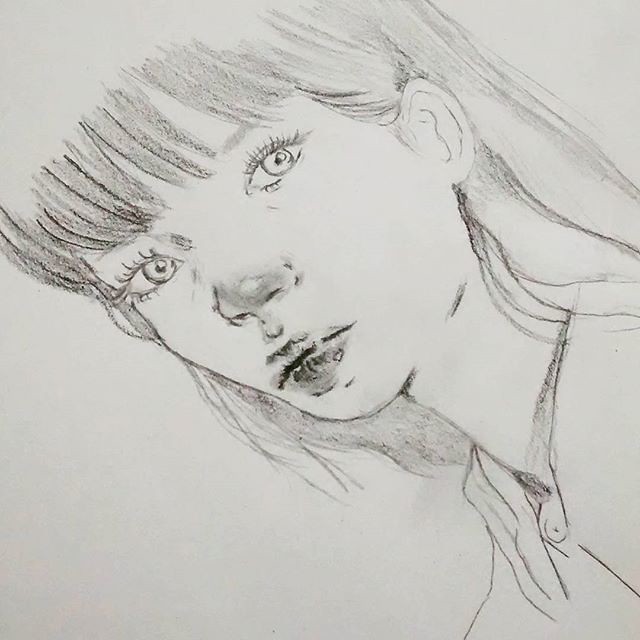This is a detailed black-and-white pencil sketch of a woman's face, drawn on a white or slightly off-white piece of paper. The sketch is cropped in a square and features the woman at a slight angle, tilted from the top left to the bottom right of the image. Her long bangs nearly cover her eyes, and her hair flows past her neck on both sides. She has light-colored eyes with long eyelashes and somewhat far-apart, circular ears. Her nose is heavily shaded at the tip, suggesting a darker or red hue. Her lips are darkly shaded in the center with lighter shading around the edges, creating a shiny appearance. The woman has a skinny neck and is wearing a collared, buttoned-up shirt with some shading around the collar area. The overall expression on her face is a blank stare.